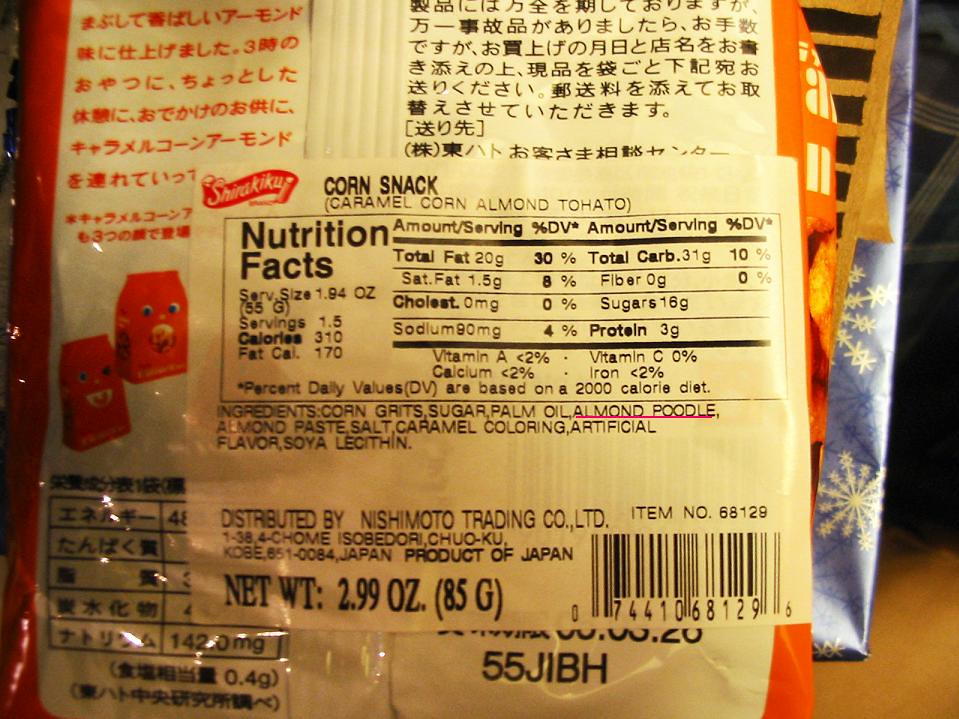This photograph features the back of a Japanese food package, specifically a corn snack labeled "Caramel Corn Almond Tohato," indicating it is a product distributed by Nishimoto Trading Company Ltd., and it is indeed a product of Japan. The packaging is adorned with Japanese characters, with black text on the right side and red text on the left, alongside playful images of smiling faces on bags. An English label with the detailed caption "corn snack, caramel, corn, almond, and tahato" along with the nutrition facts and ingredients, highlights its appeal to English-speaking markets. Notably, the nutritional information sticker includes metrics in English: 1.94 ounces per serving, 1.5 servings, 310 calories, 170 calories from fat, and 20 grams of fat per serving. The ingredients list comprises corn grits, sugar, palm oil, almond paste, salt, caramel, coloring, artificial flavors, and soya, with a peculiar entry "almond poodle" (likely a humorous mistranslation) underlined in red. This detail suggests an attempt by the consumer to highlight a potential allergen or amusing translation error.